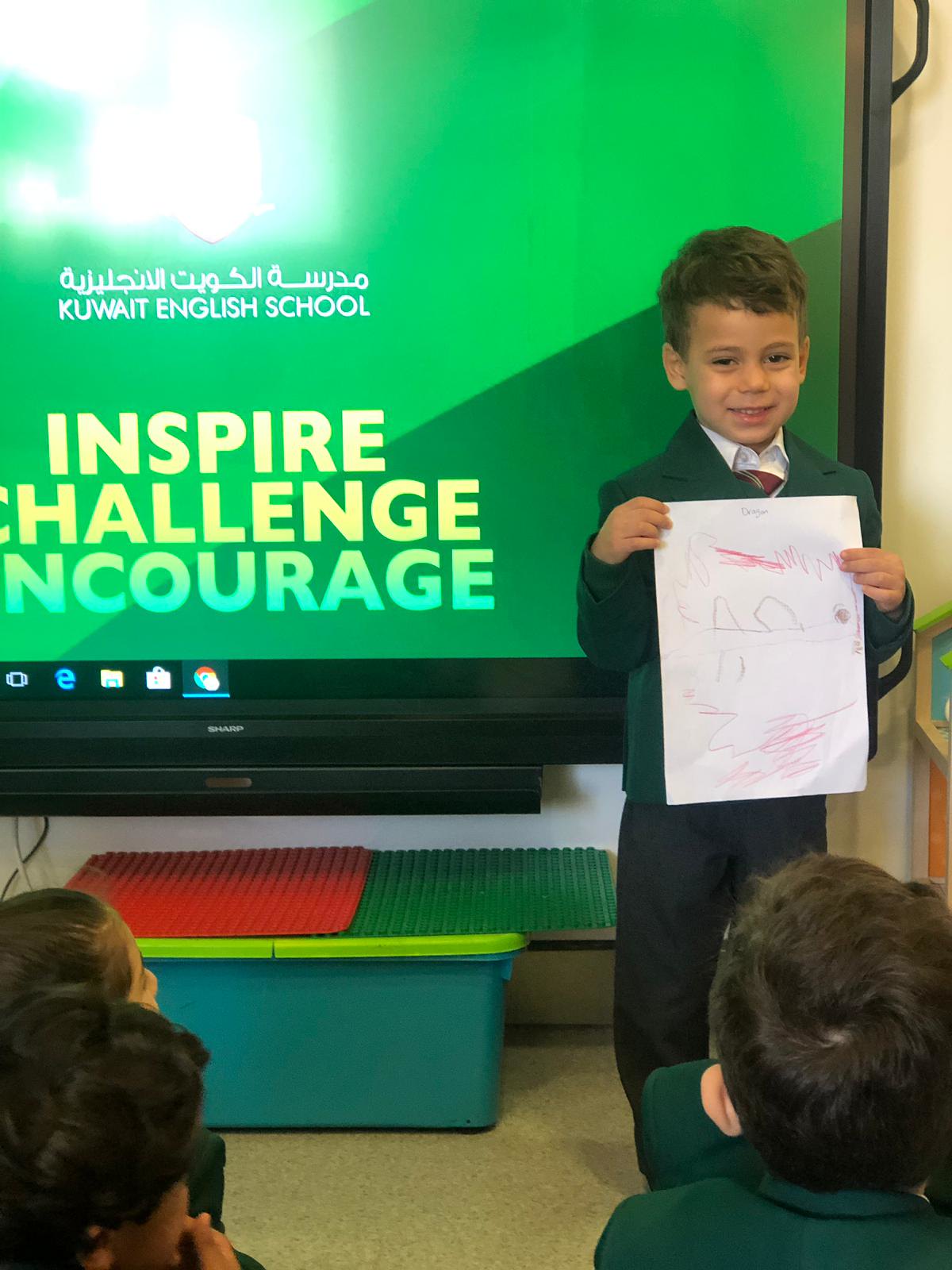In this vertical rectangular photograph, a young boy, around five or six years old, is standing confidently in front of a green board. Dressed smartly in a suit and tie with a white shirt underneath, he has short hair and is smiling warmly. To his right, the board prominently displays in white letters "Kuwait English School," and below it, in large letters, the words "Inspire" in yellow, "Challenge" in blue, and "Encourage" in light blue. The boy holds up a large piece of paper with both hands, seemingly a drawing he created, for his audience to see. Positioned in front of him, with their backs to the camera, are several other children seated and attentively listening to his presentation. Below the green board, there is a rubber container with a red and green top. The overall scene captures a moment of enthusiasm and learning in the classroom.